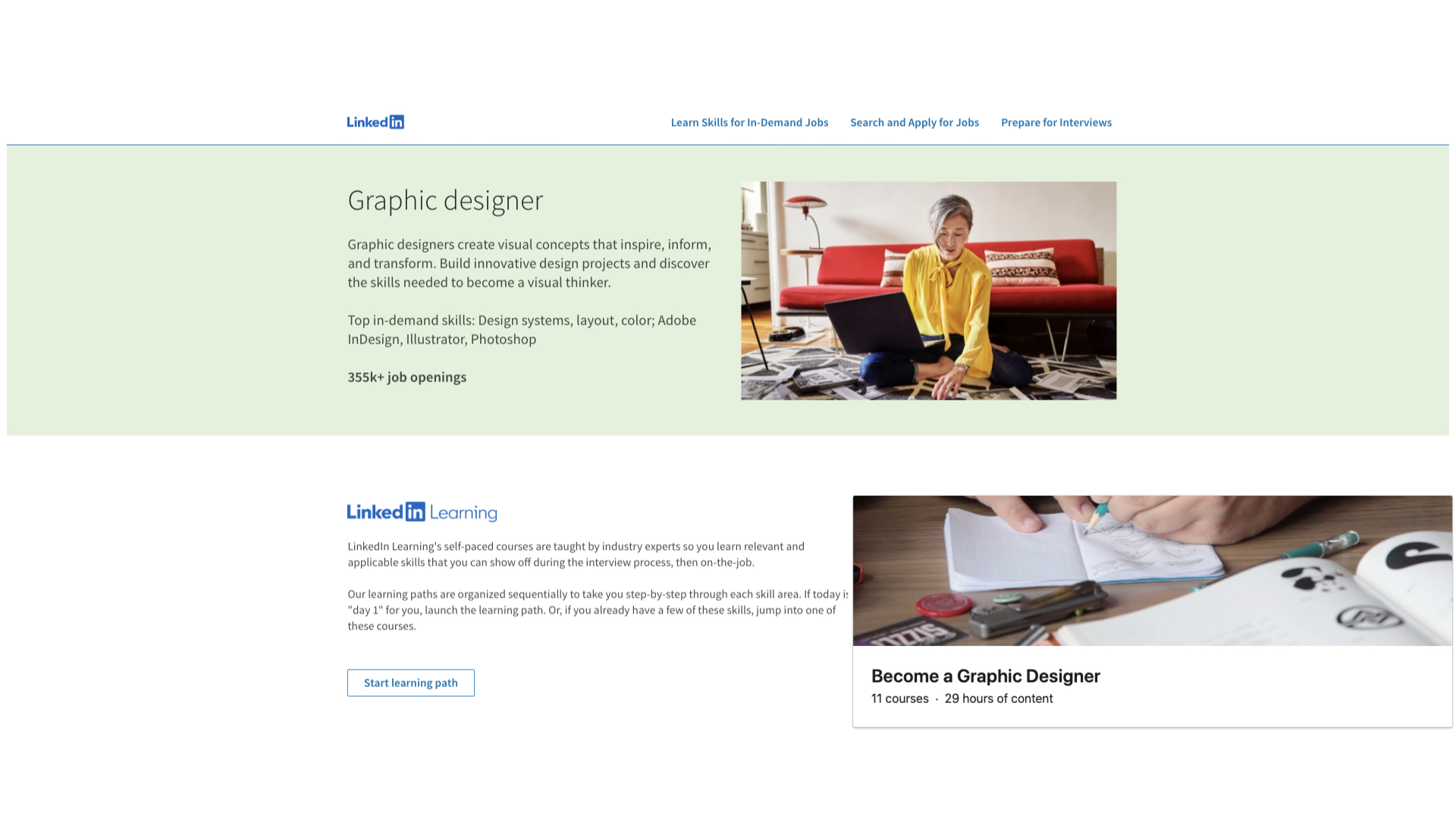The image is a screenshot from a page on the LinkedIn website. At the top of the image, "LinkedIn" is written in small blue text, and to the right, in slightly smaller blue text that reads, "Learn skills for in-demand jobs, search and apply for jobs, and prepare for interviews." 

Below this header, there is a light green seafoam colored rectangular shape containing an image of a woman. The woman is wearing a long-sleeve yellow shirt and appears to be sitting on her floor with a laptop on her knee. She is positioned on a black and white rug with a red couch visible behind her. 

To the left of the woman’s image, there is some text that reads, "Graphic Designer. Graphic designers create visual concepts that inspire, inform, and transform. Build innovative design projects and discover the skills needed to become a visual thinker. Top in-demand skills: design systems, layout, color, Adobe Design, Illustrator, Photoshop. 355K+ job openings."

Underneath this section, there is another image. This image shows someone handwriting in a small notebook, surrounded by an open book and several other small items on what is likely a desktop. To the left of this image, there is text that reads, "LinkedIn Learning," though the text further is unreadable due to the white background.